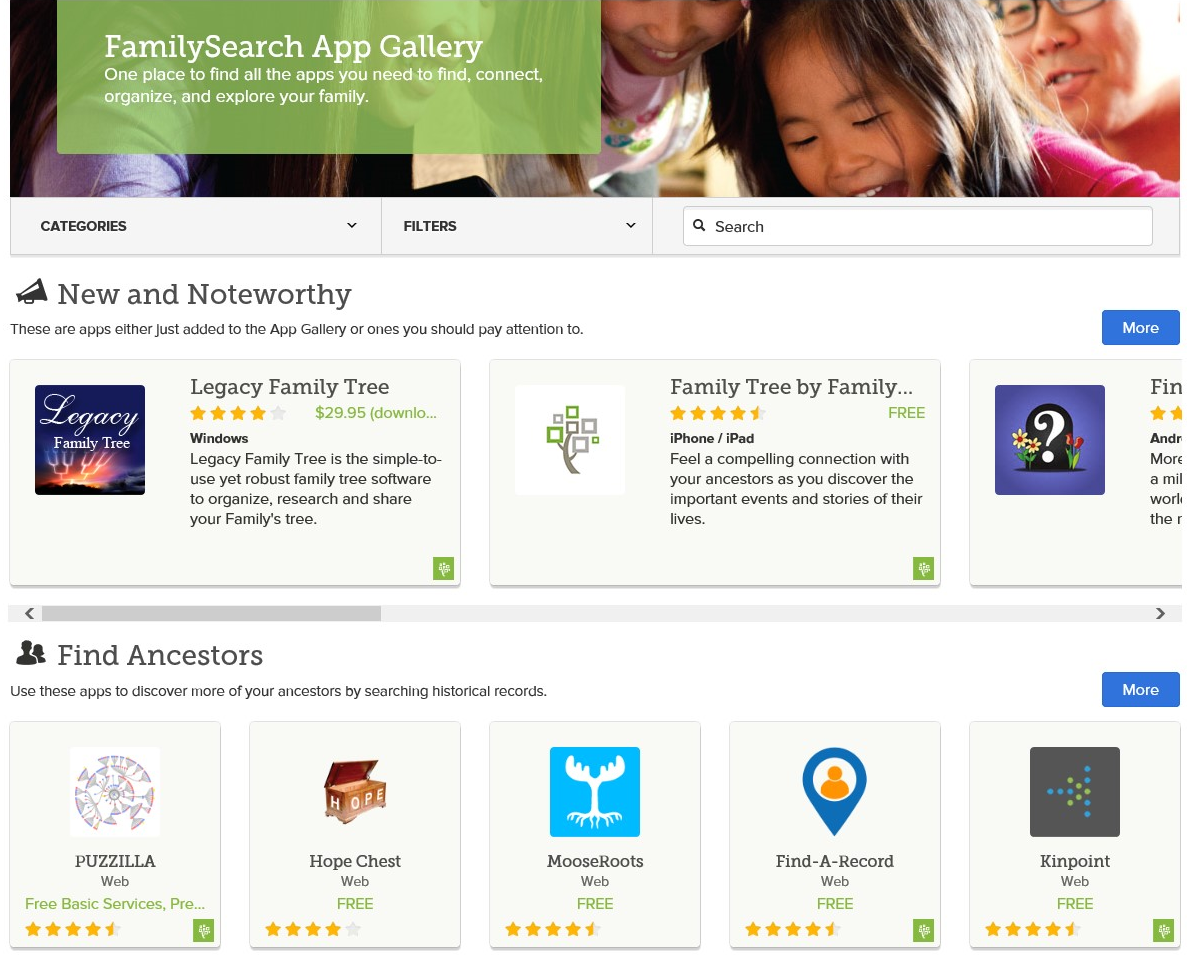The image displays a section of the Family Search App Gallery, beginning with a prominent green banner at the top labeled "Family Search, App Gallery." This banner invites users to find, connect, organize, and explore their families through various applications available in one place. Below the banner, there are options labeled "Categories" and "Filters," next to a search box for user convenience. 

Directly beneath these navigation tools, the heading "New and Noteworthy" showcases apps recently added or deemed particularly significant. Below this heading, there are detailed listings of highlighted applications:

1. **Legacy Family Tree**
   - **Rating:** Four stars
   - **Price:** $29.95
   - **Platform:** Windows
   - **Description:** A user-friendly yet comprehensive software designed to help you organize, research, and share your family tree.
   
2. **Family Tree**
   - **Rating:** Four and a half stars
   - **Price:** Free
   - **Platform:** iPhone, iPad
   - **Description:** This app enables a deep connection with your ancestors by allowing you to discover important events and stories from their lives.

Finally, the section labeled “Find Ancestors” highlights tools that can be used to uncover more information about your ancestors through historical record searches.